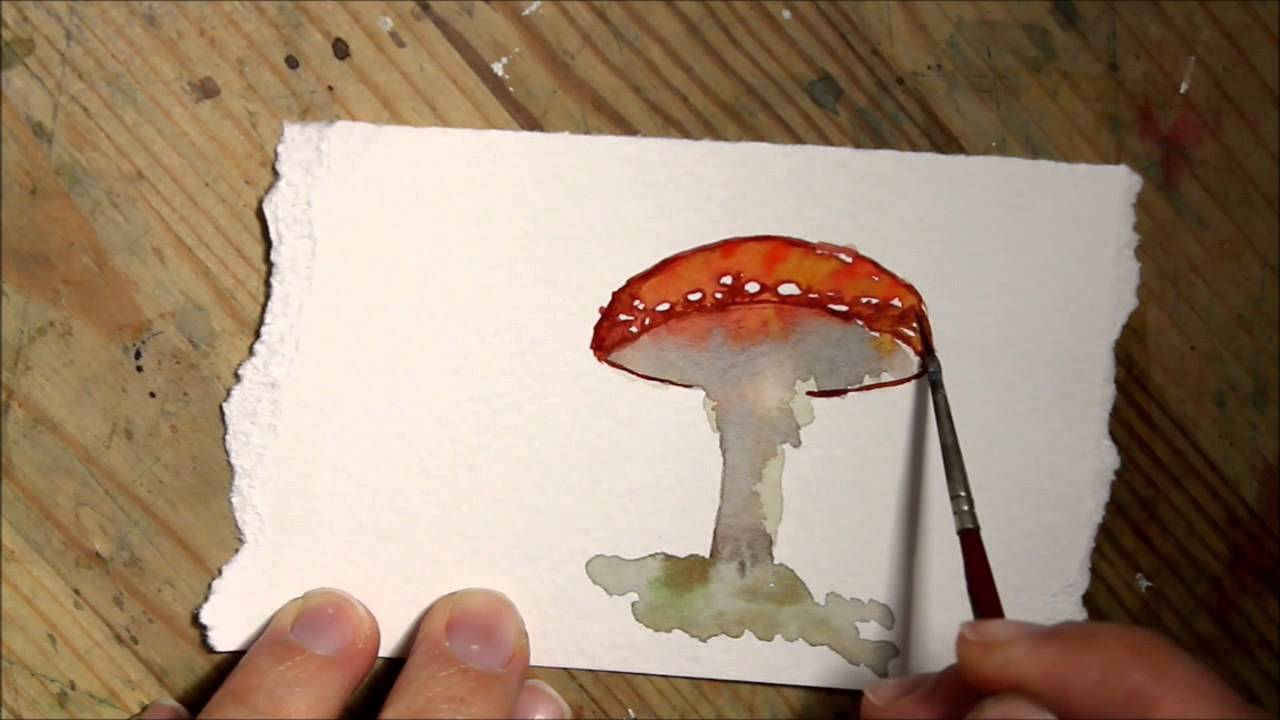The image depicts a detailed watercolor painting in progress, focused on a mushroom with a vibrant red cap dotted with white spots. The mushroom's stalk and the minimalistic ground around it are rendered in a similar white hue. This artistic creation is being crafted on a small, cut-out piece of thin white paper, which reveals uneven, torn edges, and is held firmly by the artist's left hand at the bottom left corner. The painting is set against a wooden surface, likely a table. The artist's right hand holds a brush, actively adding details to the mushroom on the right side of the paper. A soft light source from the left side of the image illuminates the scene, enhancing the rich colors and textures of the watercolor artwork.